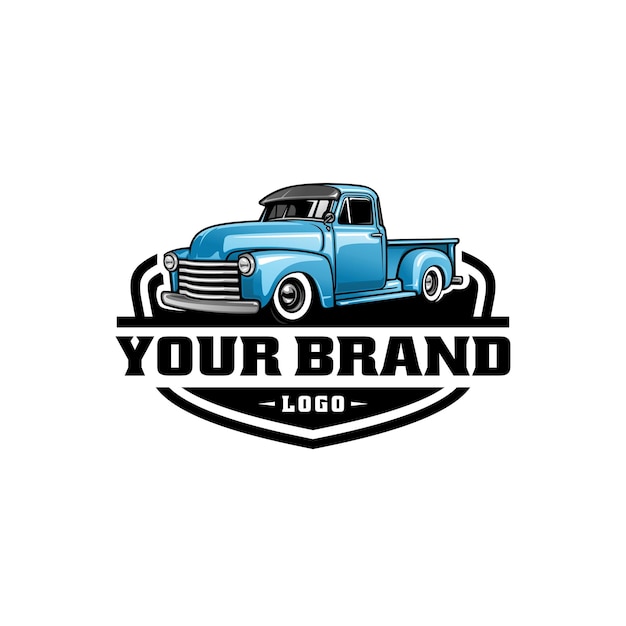This image is a stylized promotional logo set on a white background, designed as a template for advertisers to customize with their own brand. Dominating the graphic is a cartoonishly hand-drawn, vintage light blue pickup truck, reminiscent of models from the late 50s to early 60s. The truck is parked at an angle with its front facing slightly to the left, featuring a round hood, white sidewall tires with white rims, and a black visor above the windshield. The truck also includes a silver bumper and white headlights, adding to its retro aesthetic.

Beneath the truck sits a black shield-shaped emblem, outlined by a double line design. At the center of this emblem is the generic text "your brand" in black capital letters, indicating where a brand name could be inserted. Directly below this is the word "logo" in an ornate, embellished white script, flanked by two small arrows. The overall design serves as a flexible and professionally crafted template for potential advertisers to showcase their own branding.